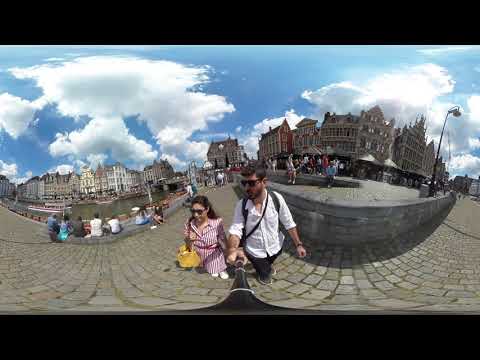A highly distorted Fish Islands photograph captures a picturesque medieval town during mid to late afternoon. The cobblestone pathway curves through the foreground, where a young couple stands. The man, who has dark hair, a beard, and wears dark glasses, a white shirt, and dark pants, holds a selfie stick, capturing their image. He has a black backpack slung over his shoulders. The woman beside him, with dark hair and sunglasses, dons a long red and white vertically striped dress and carries a yellow bag. Behind them, the scene warps whimsically, featuring curved stone buildings with spires and pathways. To the left, a river with boats flows serenely, and a couple sits on its bank, watching the activity. The sky above is a rich blue, dotted with many white, puffy clouds, completing the enchanting and surreal atmosphere of the old city.